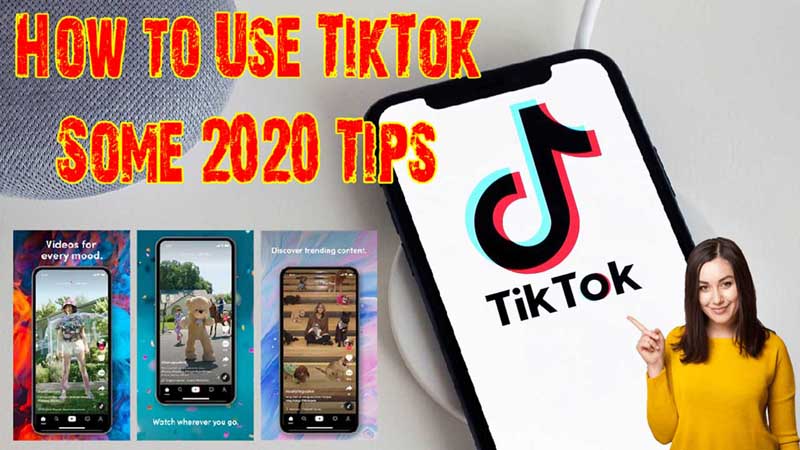The image appears to be a YouTube thumbnail with a detailed and colorful design. In the top left corner, there's a small, barely distinguishable grey fabric object resembling a Google speaker. Overlapping this, in large bold red letters with a yellow outline, the text reads "How to use TikTok: Some 2020 Tips." The "PS" in "Tips" is slightly obscured by an image of a smartphone displaying the TikTok icon and the word "TikTok" beneath it on a plain white background.

In the bottom right corner of the thumbnail, a woman with shoulder-length brunette hair, parted on the right side, is smiling and pointing towards the word "TikTok." She has light skin and is wearing a yellow jumper, although her eye color is indistinguishable.

The bottom left corner features three smaller images of mobile phone screens, each with accompanying text. The first shows someone standing in a garden with the caption "Videos for Every Mood," set against a background of blue and orange flames. The second image, against a blue background with indistinguishable elements, displays a person in a bear mascot costume standing on a street with the text "Watch Wherever You Go." The third image, which seems to show a person sitting with a possible dog beside them, has the caption "Discover Trending Content" and is set against a tie-dye background of blue and pink colors.

The main image background is grey, with a wire extending from behind the smartphone. It can be inferred that the phone rests on a wireless charger and the wire is part of this charging setup.